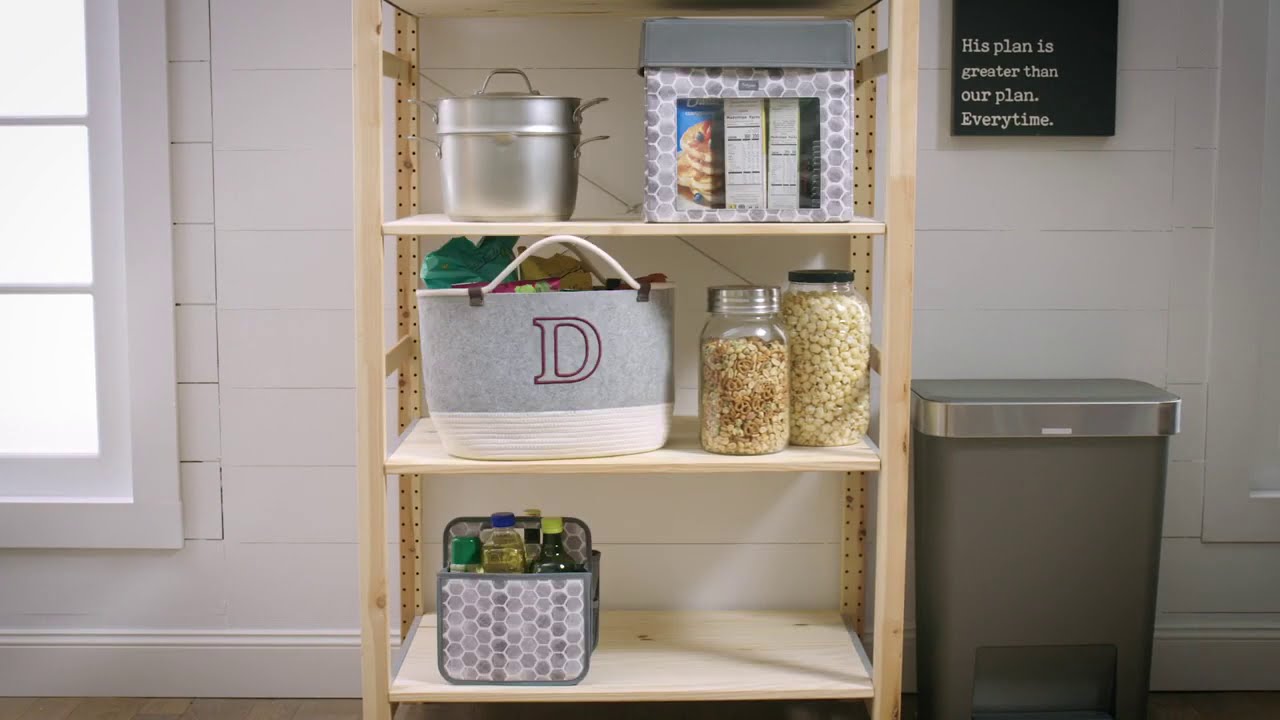In this detailed image, a light-colored wooden shelf system with three tiers is situated against a white brick wall in a kitchen. To the left, there is a wide-open window that allows natural light to flood the area. Adjacent to the shelf, on the right side, a silver trash can with a foot-operated lid stands on the floor. Above the trash can, a black poster with white text reads, "His plan is greater than our plan every time."

On the bottom shelf of the unit, a gray and white caddy holds various oils, including vegetable and olive oil. The middle shelf features a couple of large jars containing grains or cereals; one jar appears to hold pretzels or pasta. Beside these jars, a gray and white basket contains fabric or bags whose contents are not clearly visible. The top shelf holds a white and gray box with a transparent window displaying pancake mix and cereals, alongside a silver pot and a container adorned with silver hexagons. Additionally, the shelf contains a small bag marked with the letter 'D' and red markings.